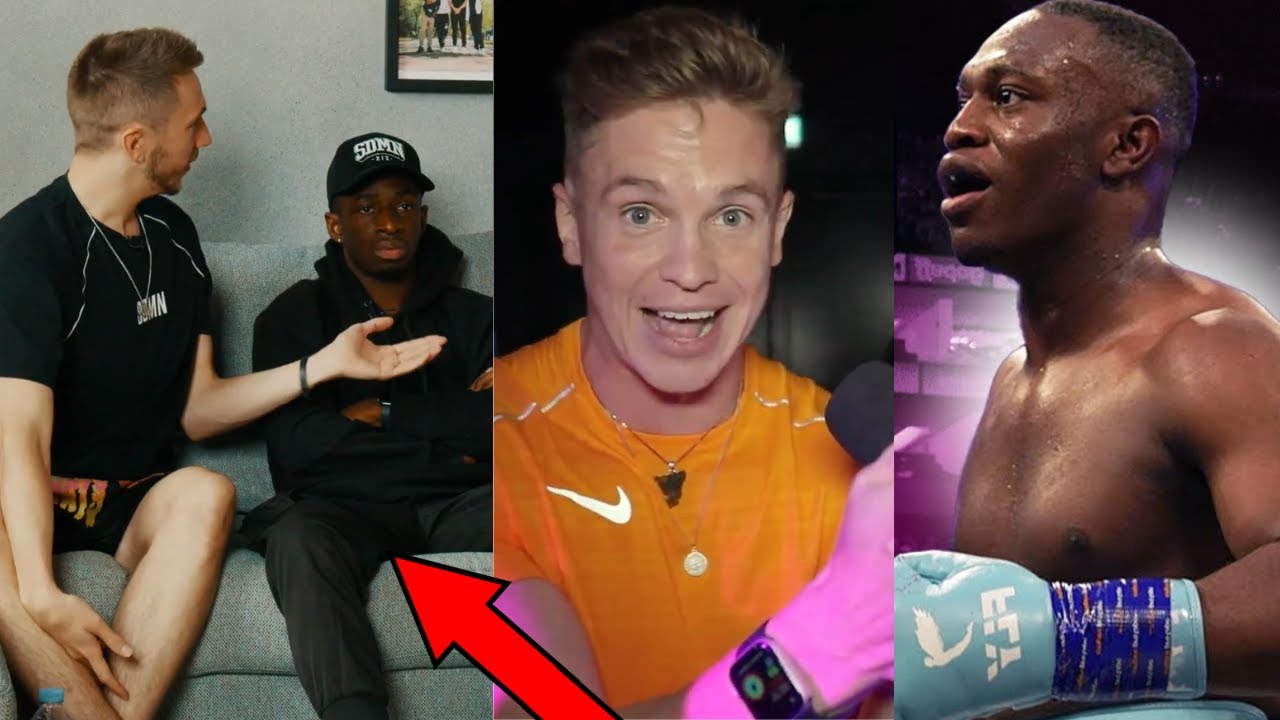On the left-hand side of the image, there are two individuals dressed in black attire. The first person, with light skin and short brown hair, is clean-shaven with a mustache. He is gesturing toward an African-American man who is wearing a black cap featuring the letters "S-D-M-N" in bold white. The African-American individual is dressed in a black sweatshirt with his arms crossed, sporting a silver watch, and matching long black pants. The individual next to him is wearing black shorts with red and yellow flame patterns. They are both seated on a dark gray couch against a matching dark gray wall. Mounted on the wall is a picture depicting four individuals: one in a black shirt and khaki pants, another in a white shirt and black pants, a third entirely in black except for his t-shirt and pants, and the last in a black vest with black pants and a t-shirt underneath. The three on the right wear white shoes, while the person on the far left is in all-black attire. A red arrow points towards the left-side image.

On the right-hand side of the image, there is a close-up of the light-skinned individual with brown hair, now wearing an orange Nike shirt with white lines around the shoulders and a white Nike swoosh to the left. He has his mouth open in an expressive manner and is looking directly at the camera. Around his neck, he sports a shark-tooth necklace and a gold necklace with a circular pendant. Beside him is an African-American man, potentially the same individual from the left image, dressed as a boxer with short, closely shaven hair. He is depicted against a purple backdrop with violet text, looking to the left with a mouthguard in place. His boxing gloves are cyan-blue with white text and feature a logo resembling a human figure with wings. The letters "YLF" are printed in white on the gloves. Additionally, the boxer’s gloves are taped with dark blue boxing tape that has orange and white text.